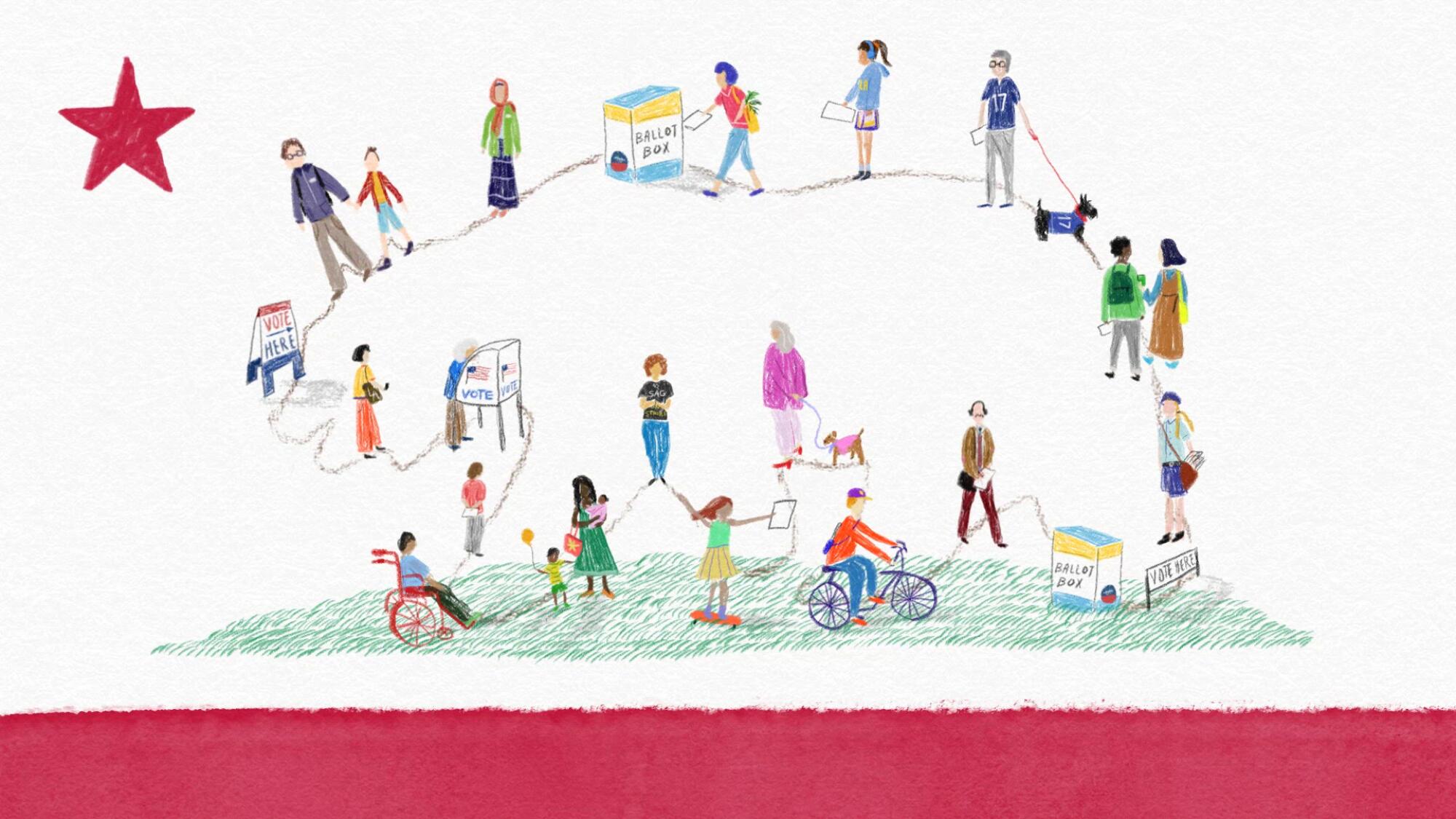This image features a hand-drawn, crayon-style artwork set against a light gray background, with a jagged pink bar along the bottom, suggesting a torn piece of paper. At the upper left corner, a prominent red star captures attention. This scene intricately depicts a diverse array of people engaged in various activities, forming a vivid and dynamic narrative.

The composition appears to take the shape of a flag, with the star potentially symbolizing a notable feature. Below, the artwork displays a continuous line of individuals, illustrating a voting process. It begins with a "Vote Here" sign, as people move towards and interact with ballot boxes, some enclosed in voting booths.

The colorful cast includes a man in a wheelchair, a woman on a skateboard, a boy on a bicycle, and a man walking a dog, all attired in a spectrum of clothing hues—blue, green, and pink tops among them. This variety emphasizes a depiction of inclusivity and democracy. The lower section transitions into a green, grassy environment, adding a touch of natural scenery.

In essence, this detailed illustration merges themes of civic duty, diversity, and communal engagement, all framed within an artistic representation reminiscent of a flag, celebrating the collective act of voting.